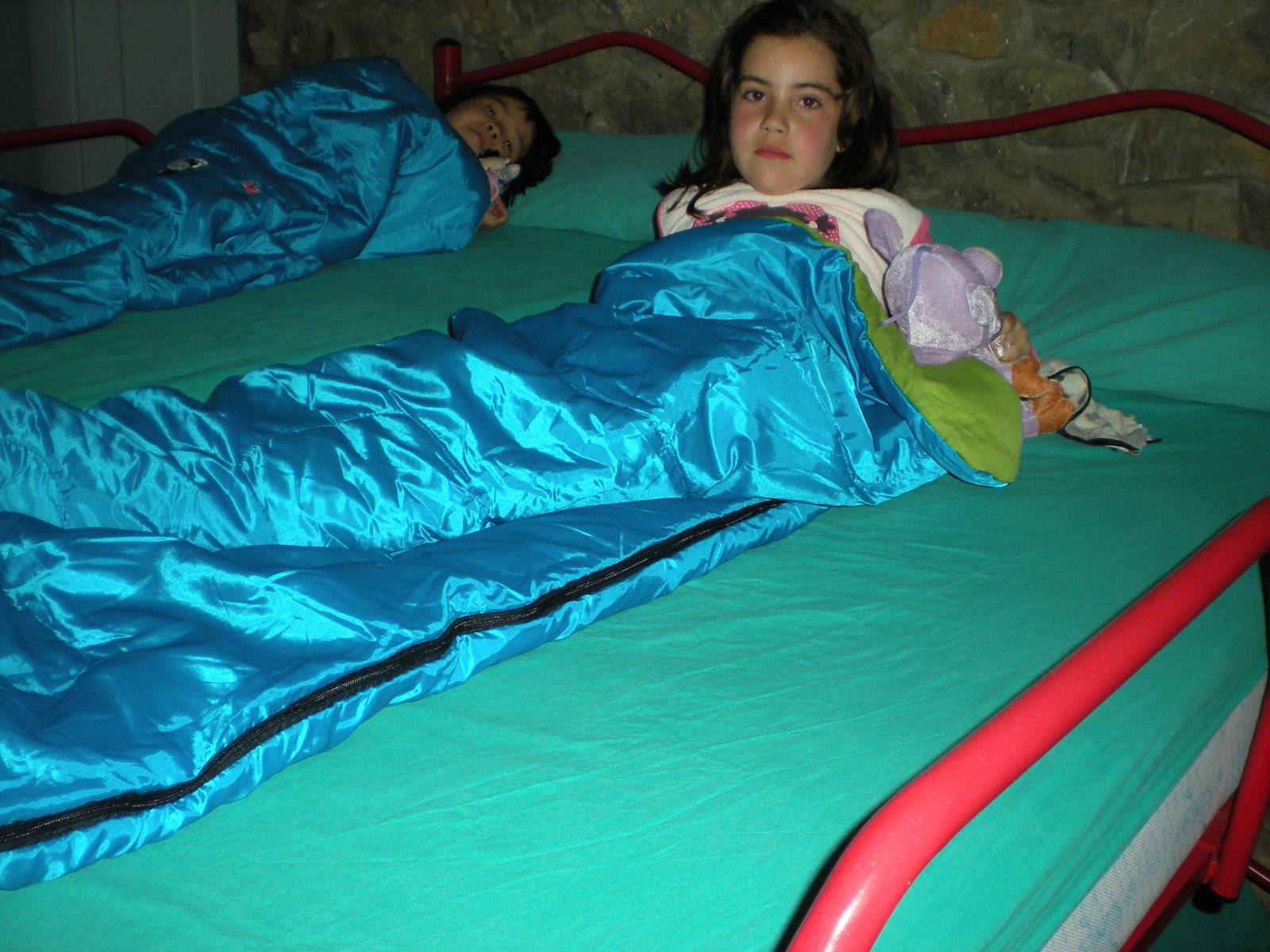This vibrant color photograph captures two young girls lying in close-proximity twin beds, adorned with bright green sheets and framed by distinctive red metal railings. Both children are snuggled into shiny, silky blue sleeping bags that gleam under the light; these sleeping bags each feature a black zipper along the right-hand side and reveal a bright, frog green interior. 

In the foreground, the girl who is more prominent in the image sits upright, gazing directly into the camera. She is wearing a sleeveless t-shirt and is accompanied by a grey stuffed animal. Her sleeping bag has eye-catching patches, and her expression is one of curiosity or engagement. Further back, the second girl appears to be smiling in her sleep, her eyes seemingly closed due to the distance and image quality. She too has a stuffed animal beside her. 

The background reveals a headboard with a green and yellow roundish pattern, and a stone-like surface accentuates the cozy setting. The pillows against the wall are encased in green pillowcases, complementing the overall color scheme of the bed area.